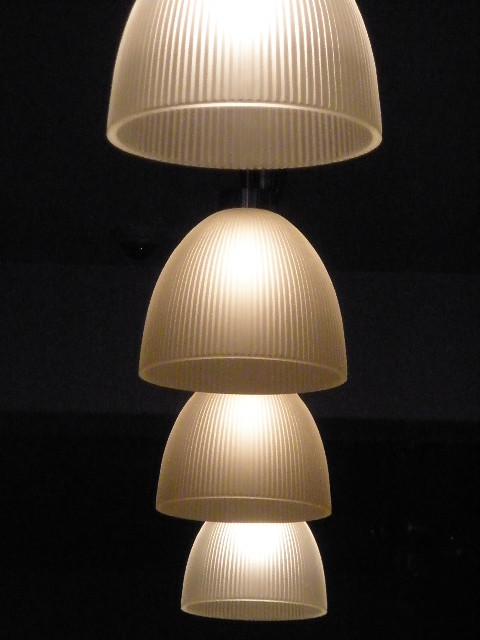This image is a digital illustration in a portrait orientation, featuring four pendant-style lampshades hanging from the ceiling. The lampshades, which are translucent and made of frosted glass, are arranged in a cascading manner, receding into the distance with each one slightly overlapping the other from the top to the bottom of the image. We are looking up at the lamps from below, giving the sense that the lamps are evenly spaced vertically. The lampshades are designed with a simple, conical shape, wider at the bottom where the light bulbs are visible, and narrow at the top, reminiscent of the top of a chicken egg. Each lampshade houses a light bulb that illuminates the interior, creating a brighter glow in the center. The second lamp from the front is suspended by a black chain link, which is subtly discernible against the pitch-black background, adding to the ethereal quality of the scene. The lampshades exhibit a ridged texture and appear uniformly smooth without any additional detailing, set against an entirely dark backdrop, capturing a minimalist aesthetic with a focus on the interplay of light and shadow.